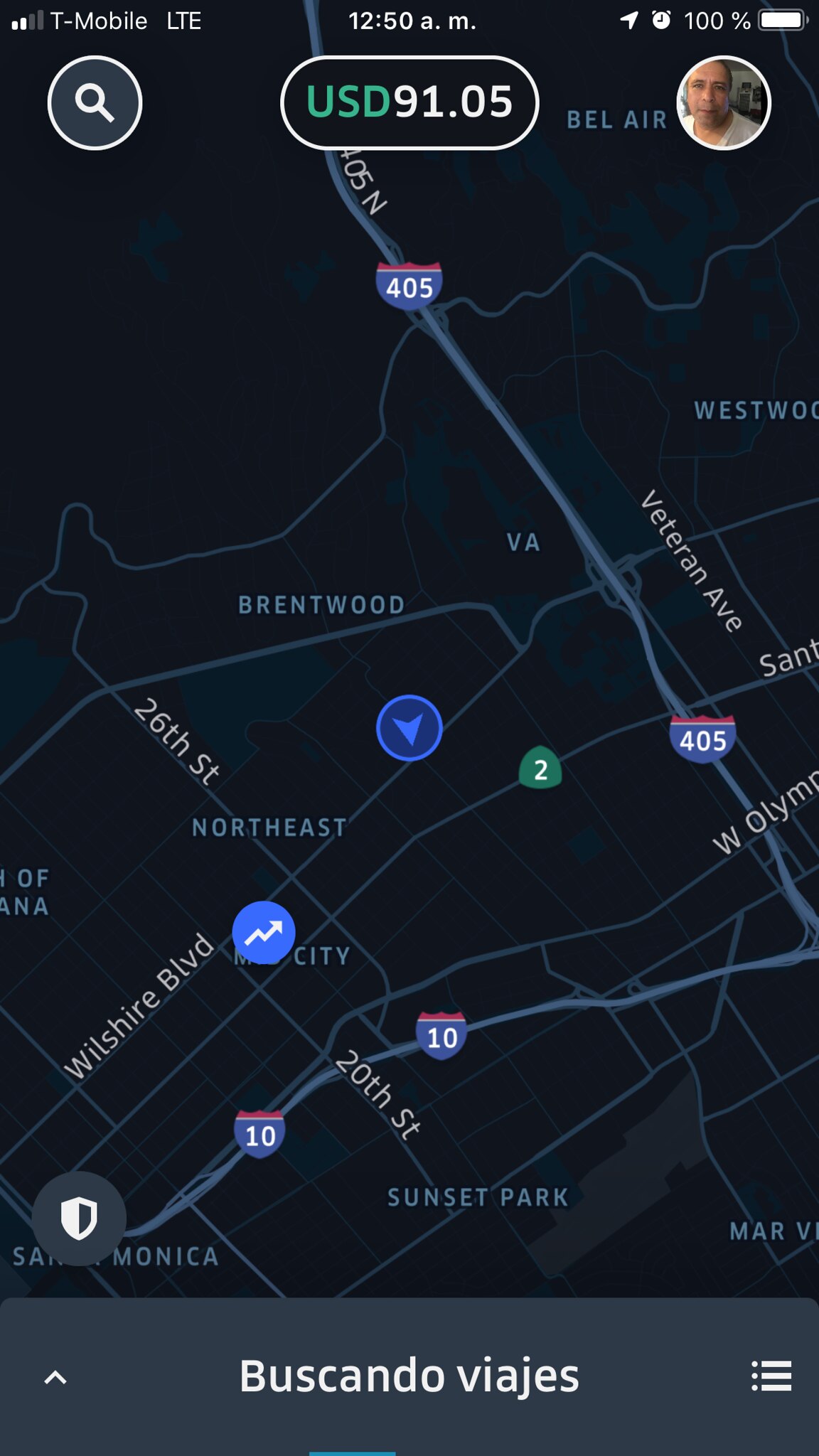This detailed caption describes a screenshot of a map displayed on a smartphone, highlighting various elements and icons featured on the screen:

---

The screenshot displays a map on a smartphone with numerous elements at the top of the screen and within the map itself. At the very top center of the screen, there's a long, oval-shaped green label with "USD" written in white letters followed by "91.05". On the upper-left corner, a circle contains an hourglass and a magnifying glass icon, and above this, it says "T-Mobile LTE". The top bar also shows the time as "12:50 AM" and further to the right, it indicates a full battery with a "100%" label next to a battery icon. Beside the battery icon, there is a clock symbol and an arrow pointing upwards towards the right. 

Below this top bar, a white circle encloses a man's face. From the center of the map, a blue line extends down towards the right, marked by an emblem with "405". The emblem resembles a shield with a blue background and the number "405" in white. Near the center of the map, there's a blue circle with a dark line containing an arrow pointing downward, adjacent to a green oval with the number "2" inside. As the blue line continues downward, it meets another blue circle with a zigzag line and an arrow pointing up towards the right. Further down, another blue line extends from the left to the right side of the map, labeled with an indicator for "Interstate 10". Below this, the map displays the area labeled as "Sunset Park" and "Northeast Brentwood".

At the very bottom of the screen, a long, dark blue bar displays the text "Piscanto Valleys". On the right side of this bar, there are three horizontal lines with dots next to them, and on the left side, there is an upward-pointing arrow.

---

This caption succinctly describes the image while providing detailed information about the various elements and their positions on the screen.